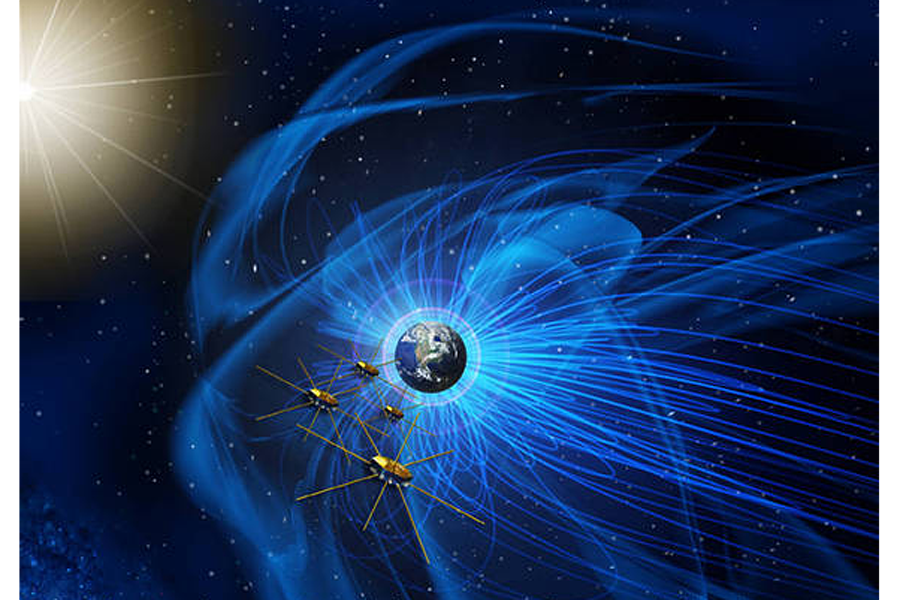A digital artwork depicts a distant view of planet Earth, positioned slightly below the center of a blue-toned space background peppered with stars and varying shades of blue. The planet, occupying about 5% of the image, is encircled by light blue lines radiating outward, particularly to the right. In the top left corner, a bright star, identifiable by its white outline and radiating beams, illuminates part of the scene. Surrounding Earth, four spider-like vessels, arranged in a clockwise formation, appear with notable size variation—the largest is near the middle right, followed by progressively smaller ones, with the smallest next to it and the second-largest below the smallest. These vessels, with their long protrusions, seem closer to the viewer than the Earth, adding a complex layer of depth to this cosmic tableau.